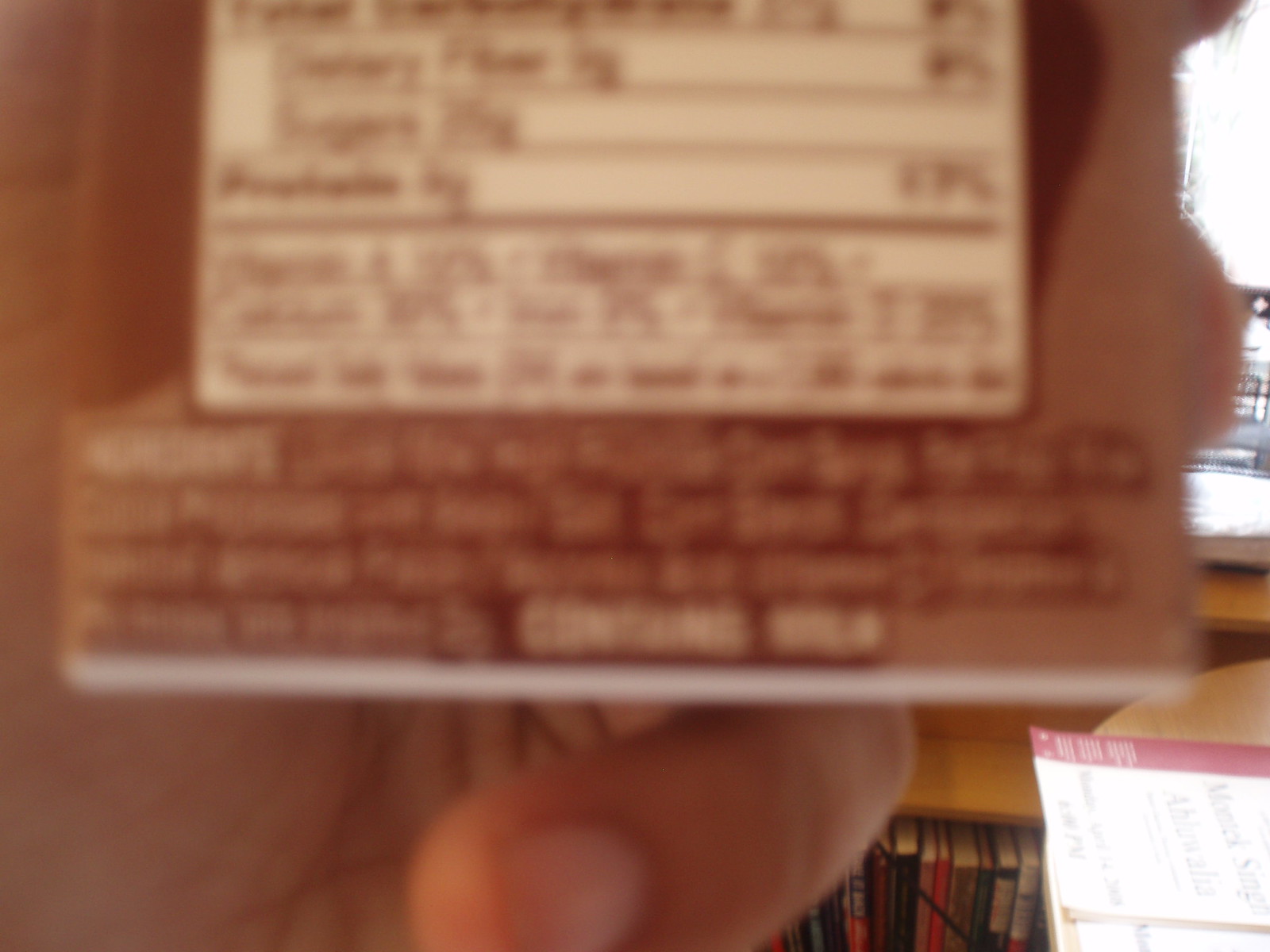In this blurry close-up photograph, a light-skinned man is holding a brown-packaged item by its back, facing the camera. His hand is prominently featured, obscuring most of the package. The visible but unreadable white nutrition label shows sections for sugars and proteins, while the bolded text "contains milk" is discernible at the bottom. The background reveals part of a low bookcase filled with books and a round brown wooden table adorned with white and purple papers.